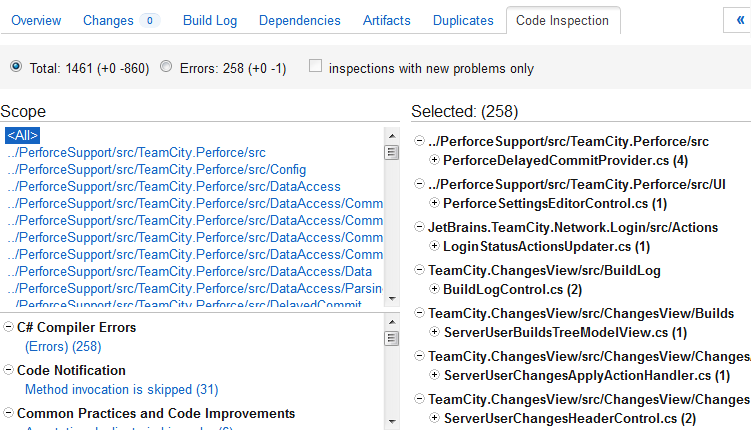The image appears to be a screenshot from a code inspection tool, showcasing a detailed overview of a coding project's analysis results.

At the top of the image, the heading "Code Inspection Overview" is prominently displayed. Directly beneath it, a navigation bar containing various tabs is visible: "Overview," "Changes," "Build Log," "Dependencies," "Artifacts," "Duplicates," and "Code Inspection," with the current view set to "Code Inspection."

Below the navigation bar, summary statistics are presented. The first line indicates:
- Total lines of code: 1461 (with no recent additions or deletions)
- Errors: 258 (with no new additions or one less than before)
- Inspections with new problems: None currently unchecked

Further down, there's a section labeled "Success Scope," followed by detailed lines of code, which are not fully visible in the image.

A section named "Compiler Errors" reports:
- Total errors: 258
- A specific notification: "Method invocation is skipped 31 times due to common practices and code improvements," with some details cut off by the image's frame.

The image highlights that 258 errors have been selected for review. A list follows, presumably detailing each coding error by line number, though this list is not expanded in the visible screenshot.

In essence, this screenshot captures a code inspection tool's interface, designed to help developers identify, review, and correct errors within their codebase.